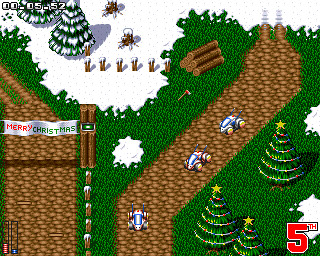The image depicts a festive, snowy scene set in a video game. On the right side, large text displays "5TH" with the "TH" positioned at the top of the number five. To the left, a banner reads "Merry Christmas." The landscape features a brown road, surrounded by green patches of grass, and partially covered in snow. At the top left corner, a video timer reads "00:05-52."

Scattered throughout the scene are various elements that add to the wintery atmosphere. Snow-covered pine trees stand tall, and there is a noticeable pile of logs on the right side. An axe lies on the ground nearby, hinting at recent activity. A decorated Christmas tree stands proudly at the bottom right, adorned with red ornaments and strings of lights, and crowned with yellow stars.

A white car, distinctive with blue, bunny-like ears and yellow wheels, adds a whimsical touch. Behind this vehicle, tire tracks trace into the snow at the top right of the image. In the background, another car can be seen further back in the scene. At the bottom left, two bars are displayed, one filled with red and the other with blue, perhaps indicating in-game statistics or health levels.

The blend of festive decorations, vehicles, and snowy details creates an immersive, holiday-themed gaming environment.